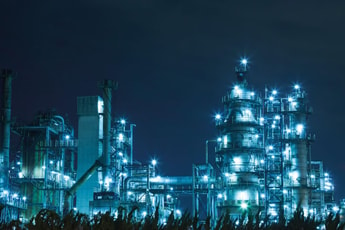The image captures a nighttime cityscape dominated by a rich, dark blue sky that lightens slightly toward the middle. At the bottom, silhouettes of trees or bushes create a stark contrast against the dark sky. The scene features a series of tall, mill-like buildings with a significant presence on the right side, highlighted by a spiral structure adorned with bright white lights, which emit a bluish hue in the darkness. Adjacent to this is a network of shorter, factory-like buildings connected by pipes and potentially stairs, all illuminated by similar white lights that also take on a light blue tint. The composition creates an atmosphere where the intense blue tones of the sky and lights interweave, painting a serene yet industrial nighttime portrait.